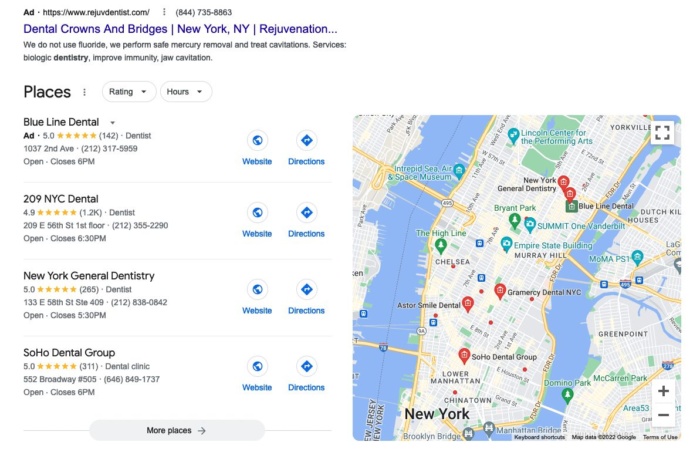**Detailed Caption:**

The image depicts a search results page likely for dental services within New York, NY. At the top of the page, there's an "Ad" label followed by a web address that begins with "HTTPS." Adjacent to this on the right is a vertical trio of dots, serving to separate the address from the subsequent information.

Below this top section, a phone number appears alongside keywords such as "dental," "crowns," and "bridges." Each segment is divided by vertical lines. Further down, there's a designation for "New York, New York," and "rejuvenation," which are also separated by lines and end with an ellipsis.

The next section is labeled "Places," featuring two oval buttons titled "Rating" and "Hours," both equipped with drop-down arrows for further interactions. 

Beneath this, listed in individual rows are several dental practices: "Blue Line Dental," "209NYC Dental," "New York General Dentistry," and "Soho Dental Group." Each row contains icons for "Website" and "Directions," along with ratings, addresses, hours of operation, and phone numbers.

On the right-hand side of the image, there's a map with red dots marking the locations of these dental practices. For instance, a red dot near Lower Manhattan indicates the location of "Soho Dental Group." Similarly, other red dots denote the locations of "New York General Dentistry" and additional practices, as indicated by corresponding labels on the map.